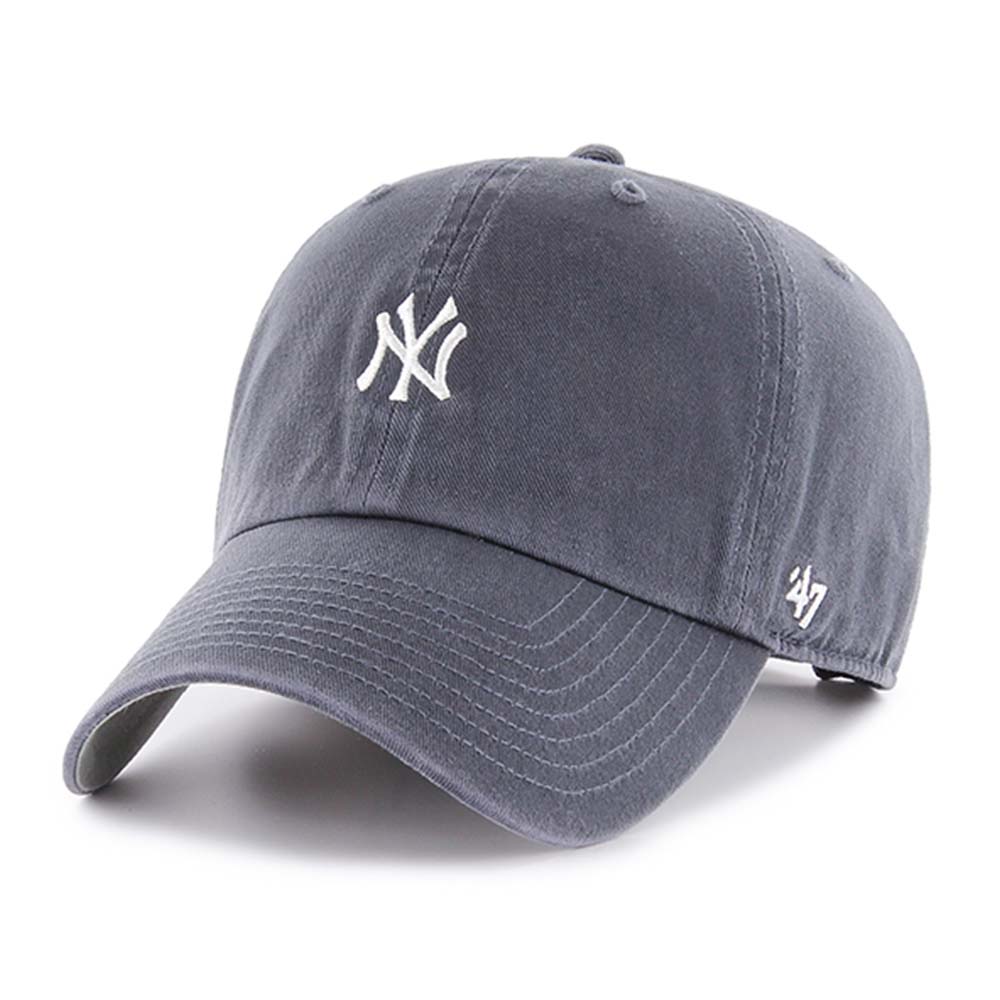The image features a light gray New York Yankees baseball cap, centrally positioned against a plain white background. The cap prominently displays the iconic "NY" logo in white lettering on the front. On the side, you can see the number "47," also in white. The material appears to resemble denim, with a texture akin to jeans. The brim is oriented towards the bottom left of the image, casting a gray shadow onto the white backdrop. Characteristic elements such as the button on top, the seams, and the riveted ventilation holes are all visible, adding to the detailed structure of the cap.